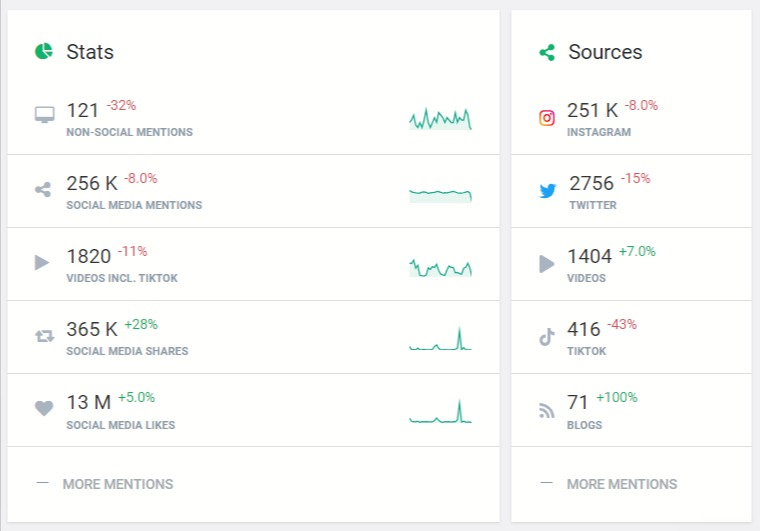The image presents a detailed statistical overview of social media metrics and mentions, organized into distinct categories. At the very top left corner of the image, the word "STATS" is prominently displayed next to a green circle. Beneath "STATS," various categories are outlined with corresponding data:

1. **Non-Social Mentions**:
   - **121** mentions, with a decrease of **32%** shown in red.
   - Accompanied by a small graph with green lines indicating trends.

2. **Social Media Mentions**:
   - **256K** mentions, with a decrease of **8%**.

3. **Videos Include TikTok**:
   - **1820** mentions, with a decrease of **11%**.

4. **Social Media Shares**:
   - **365K** shares, showing an increase of **28%**.

5. **Social Media Likes**:
   - **13M** likes, indicating an increase of **5%**.

A small note at the very bottom left prompts, "More Mentions."

On the right side of the image, starting from the top right, the word "Source" is listed, followed by detailed breakdowns of mentions across different platforms:
- **Instagram**: **251K**
- **Twitter**: **2756**
- **Videos**: **1404**
- **TikTok**: **416**
- **Blogs**: **71**

The layout is methodically organized with statistical data and trend indicators, offering a comprehensive summary of social media interactions and activity.